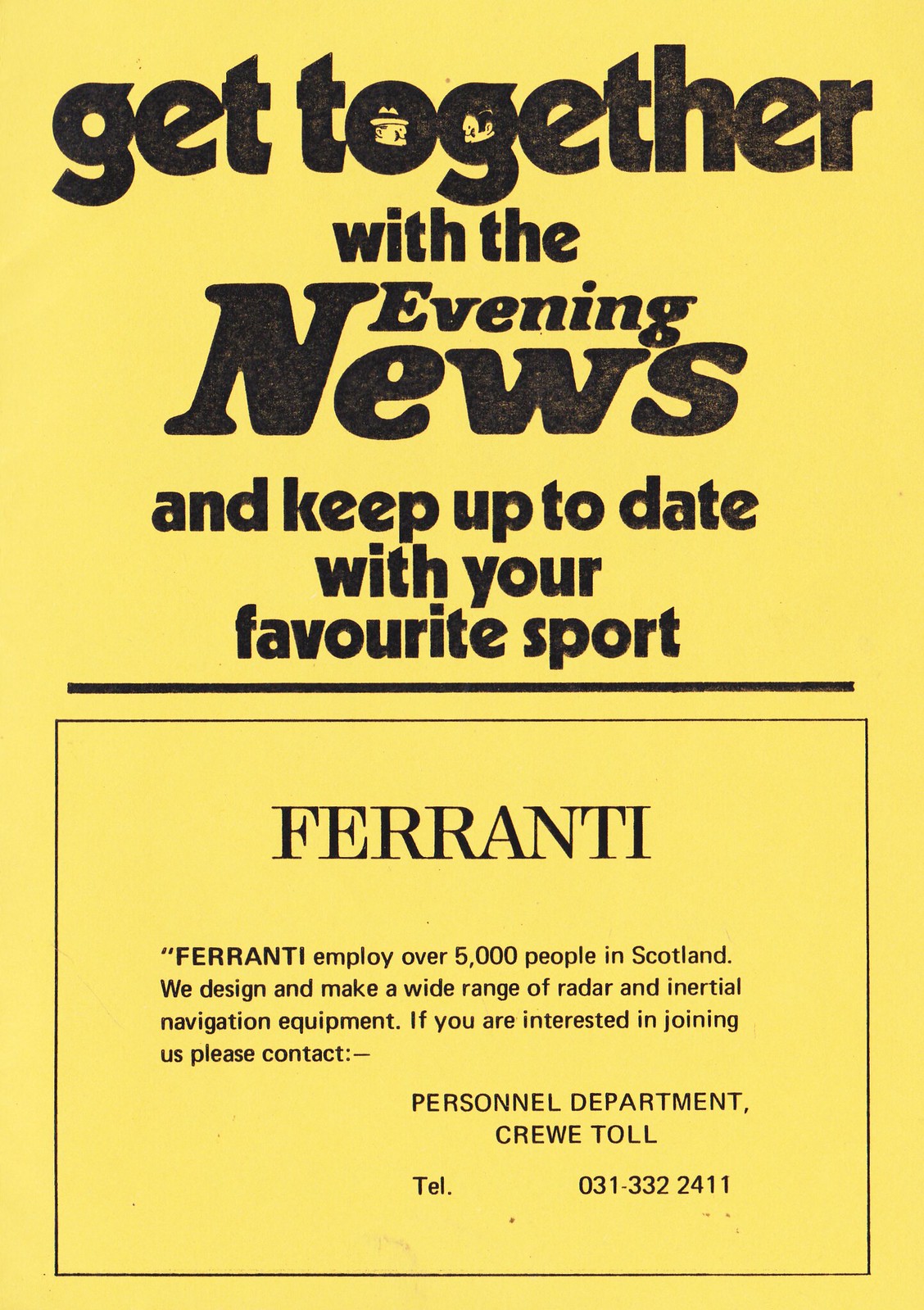This image is an advertisement with a yellow background and black text. At the top, the ad reads "Get together with the evening news and keep up to date with your favorite sport." Below that, it features a block of text within a black rectangle that prominently displays the name "Ferranti." The text continues to say, "Ferranti employs over 5,000 people in Scotland. We design and make a wide range of radar and inertial navigation equipment. If you are interested in joining us, please contact the personnel department, Crew Toll, Telephone 031-332-2411." The overall design appears to resemble a newspaper or magazine help-wanted ad, with a clean and straightforward layout.